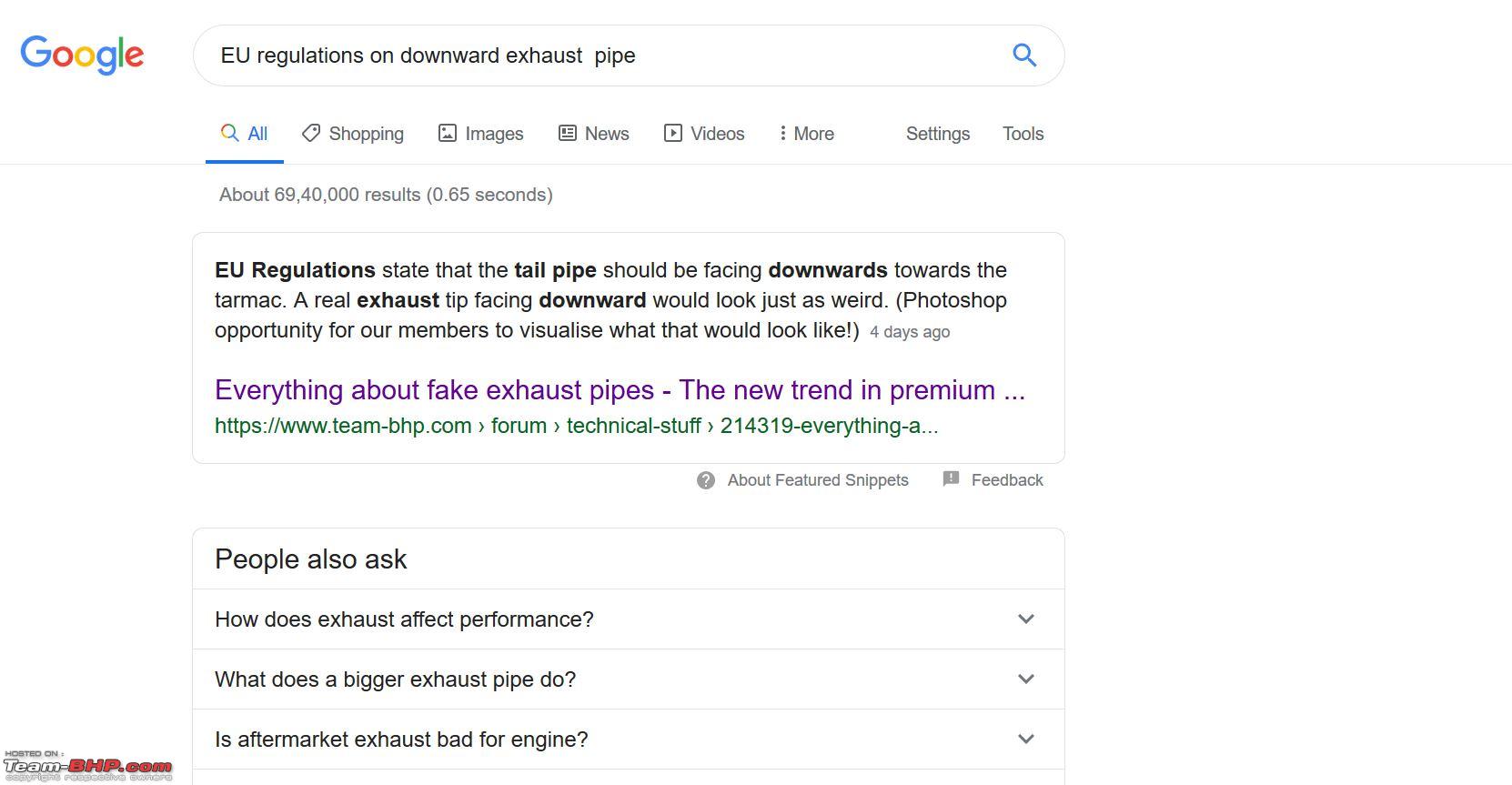In the image, a detailed Google search results page is displayed. The search query entered is "EU regulations on downward exhaust pipe." The active tab is "All," but other available tabs include "Shopping," "Images," "News," "Videos," and additional settings and tools. The iconic Google logo is visible in the upper left corner of the page.

Below the search bar, the page indicates around 69 million results, although there appears to be a discrepancy with the displayed number. The first search result is a description from the website team-bhp.com under the forum section titled "Technical Stuff." The site elaborates on EU regulations, stating that exhaust tailpipes should be directed downwards towards the tarmac, and mentions a Photoshop opportunity for users to visualize the appearance of downward-facing exhaust tips. It also briefly touches on the emerging trend in premium vehicles featuring these exhaust designs.

Further down, the "People also ask" section includes related questions such as "How does exhaust affect performance?", "What does a bigger exhaust pipe do?", and "Is aftermarket exhaust bad for the engine?" Each question is clickable, allowing users to expand and view detailed answers.

The background of the page is predominantly white, with black text used for the various search results and headings, maintaining Google's clean and simple aesthetic.